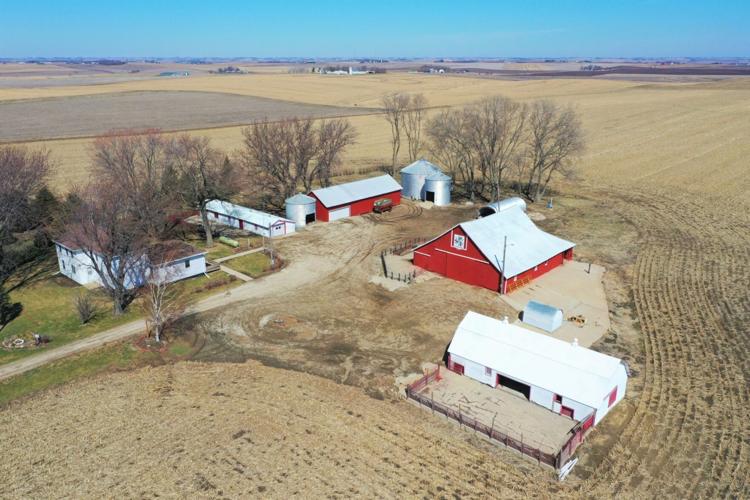The aerial view captures a sprawling farm in a remote area, transitioning from winter to spring. At the heart of the image, a prominent red barn with a white sloped roof stands out, surrounded by various farm buildings and fields. Directly below and to the right, a stable-like white structure features a sloped roof and a corral in front. To the left, partially obscured by a tall tree with barren branches, a two-story white house with a red roof is visible, hinting at where the occupants reside. Nearby, a long, narrow white building with a sloped roof and a wide garage door catches the eye, adjacent to a silver silo with a circular, spiraled roof. Behind this, a smaller red building with a significant white door and a metal roof peaks out. The landscape reveals wide expanses of flat, brown farmland with hints of budding lavender flowers and a strip of blue sky at the top, suggesting the changing seasons. In the background, fields stretch out towards the horizon, with glimpses of another potential farm.